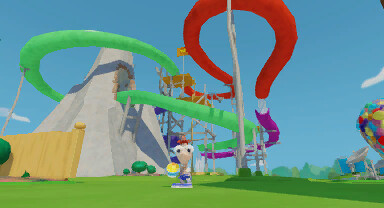In this screen capture, we see a whimsical character that appears to be from a TV show, cartoon, or video game. The central figure is a small, teardrop-shaped being with disproportionately large, flat feet clad in blue shoes. Its head is an upside-down triangle topped with a tiny cowboy hat, giving it a quirky and endearing appearance. The character's expressive black eyes gaze directly at the viewer while it holds a colorful ball, which is yellow, blue, and white. Behind this charming creature, there is a large amusement park attraction, likely a water slide, that winds through a cement mountain, adding a dynamic and adventurous backdrop to the scene. The image perfectly captures a moment filled with whimsy and fun, characteristic of animated or game settings.